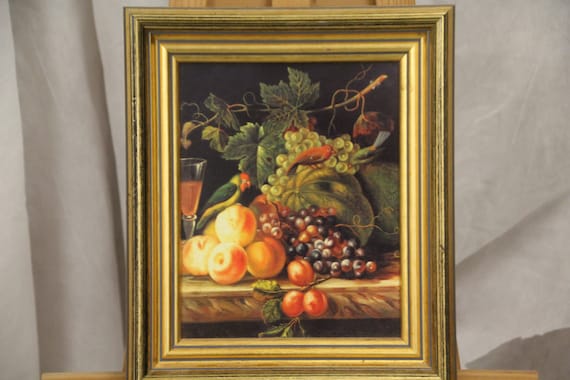The image depicts a picturesque still life painting showcasing a bountiful arrangement of fruits, including grapes, peaches, and apples, adorned with green leaves from a grape vine. A red bird is perched on the cluster of grapes, while another bird, with a red head and green body, adds a vibrant touch to the scene. To the left, a tall, thin crystal glass holds a red beverage, enhancing the elegant composition. The backdrop of the painting features a subtle gray draped surface, providing a neutral contrast to the colorful display. The artwork is encased in a luxurious, multi-layered gold frame with slightly green outer edges, further accentuating its classical appeal. The overall setting suggests an indoor environment used to photograph and possibly sell this detailed and aesthetically pleasing still life painting.